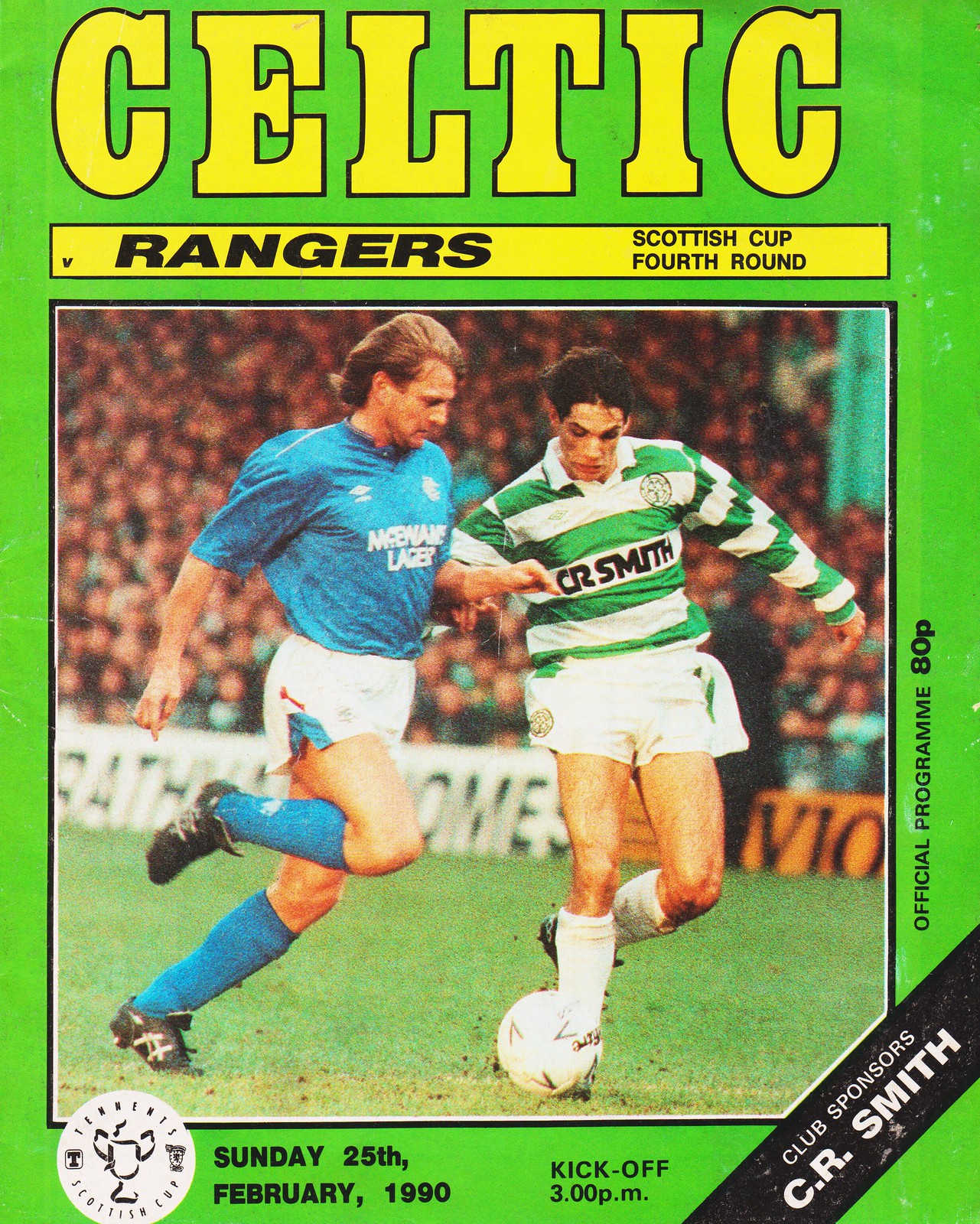This image is the cover of an official program for an English football match between Celtic and Rangers in the Scottish Cup fourth round. The cover features a lime green background with yellow and black text. At the top, "Celtic" is prominently displayed in yellow text with a black outline, and below it, within a yellow banner also outlined in black, the words "Rangers Scottish Cup fourth round" are written. Central to the cover is a photograph, bordered in white and black, depicting two football players in action on the field. The player on the left is wearing a blue soccer shirt, white shorts, and blue socks, while the player on the right has a green and white horizontally striped soccer shirt, white shorts, and white socks. A large audience of spectators can be seen in the background, emphasizing the professional nature of the event. The ball in play is white with black panels. At the bottom of the cover, the details state: "Sunday, 25th February 1990, kickoff 3 p.m. Club sponsors: C.R. Smith. Official program 80 pence."